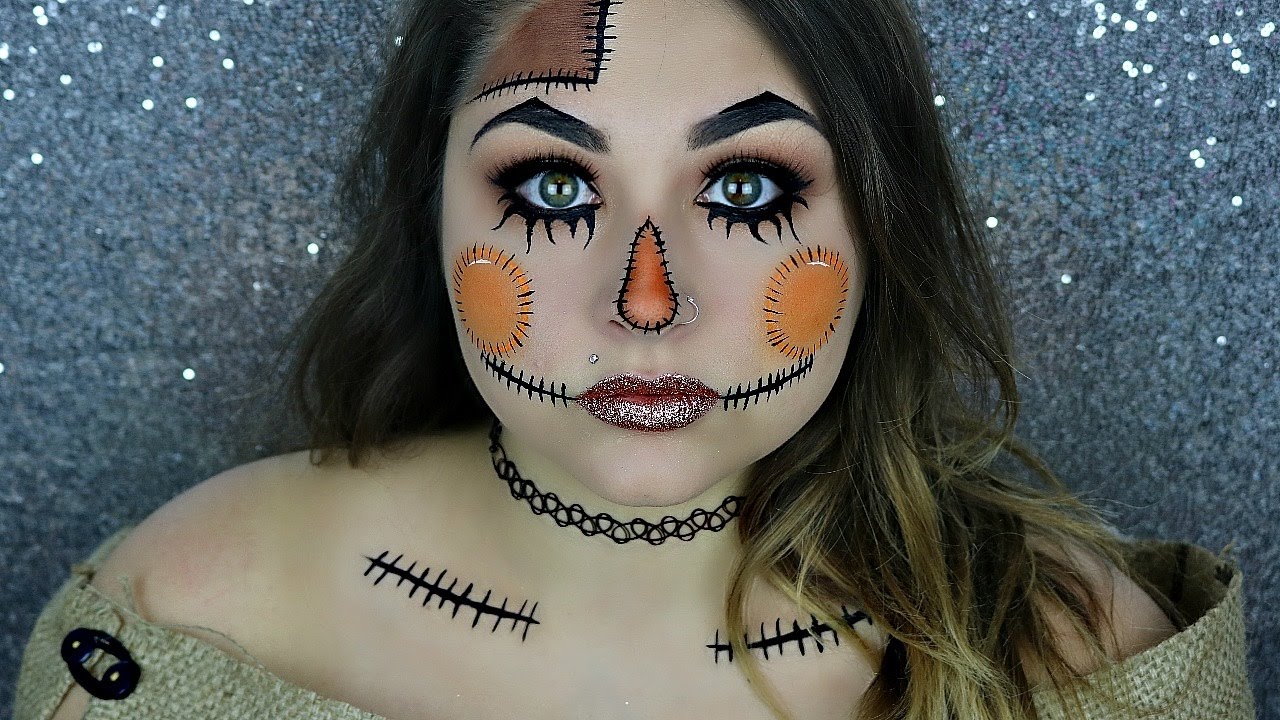The image displays a young woman with elaborate Halloween makeup against a silver, sparkly background. Her fair skin contrasts with her brown hair, which transitions into lighter shades at the ends. The makeup transforms her into a costume scarecrow: a brown patch resembling burlap is painted on the upper left side of her forehead, with black lines indicating stitching. Her eyebrows are thick, dark, and sharply angled, complementing the dramatic eyeliner extending in flare-like patterns from her lower eyelids. Her nose is painted a vivid yellow with faux stitches, and her cheeks feature two orange dots also designed to appear sewn-on. Red glitter adorns her lips, which have black stitched lines extending from each corner. She wears a black choker and additional black stitching is painted along her collarbones. Silver glitter accents her hair, adding to the overall glamorous and eerie effect. The detailed costume makeup is intricate, with each component aimed at creating the image of a whimsical, yet haunting scarecrow.